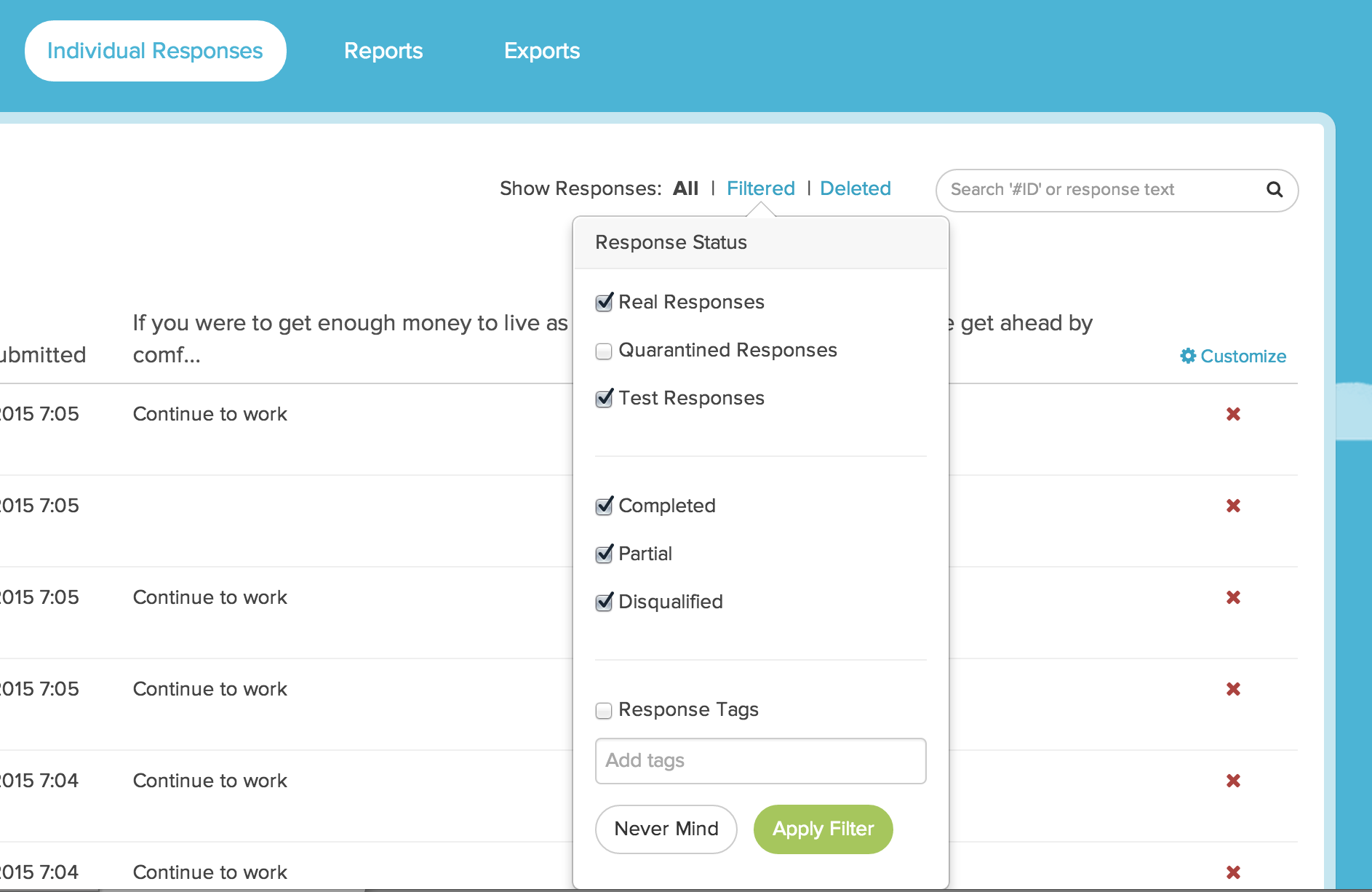**Caption:**

The screenshot displays an application or website interface with a prominent light blue banner at the top and a narrower light blue bar running down the right side. In the top left corner of the top banner, there are three selectable options: "Individual Responses," "Reports," and "Exports." The "Individual Responses" option is currently selected and highlighted by a white oval, with its text in light blue, while "Reports" and "Exports" are displayed in white.

Below the top banner, the interface features a segment titled "Show Responses," offering four filtering options: "All," "Filtered," "Deleted," and a search bar to the right. The word "All" is bold black, while "Filtered" and "Deleted" are in teal or light blue and all three are separated by small black lines. A drop-down menu extends from the "Filtered" option, labeled "Response Status," presenting several checkboxes:

1. "Real Responses" (checked)
2. "Quarantined Responses" (unchecked)
3. "Test Responses" (checked)
4. "Completed" (checked)
5. "Partial" (checked)
6. "Disqualified" (checked)

There is also a checkbox labeled "Response Tags" (unchecked) with an input field below it that says "Add Tags." At the bottom of the drop-down menu, two buttons are displayed: a white button labeled "Nevermind" and a green button labeled "Apply Filter." The results of the search are visible behind this filter menu.